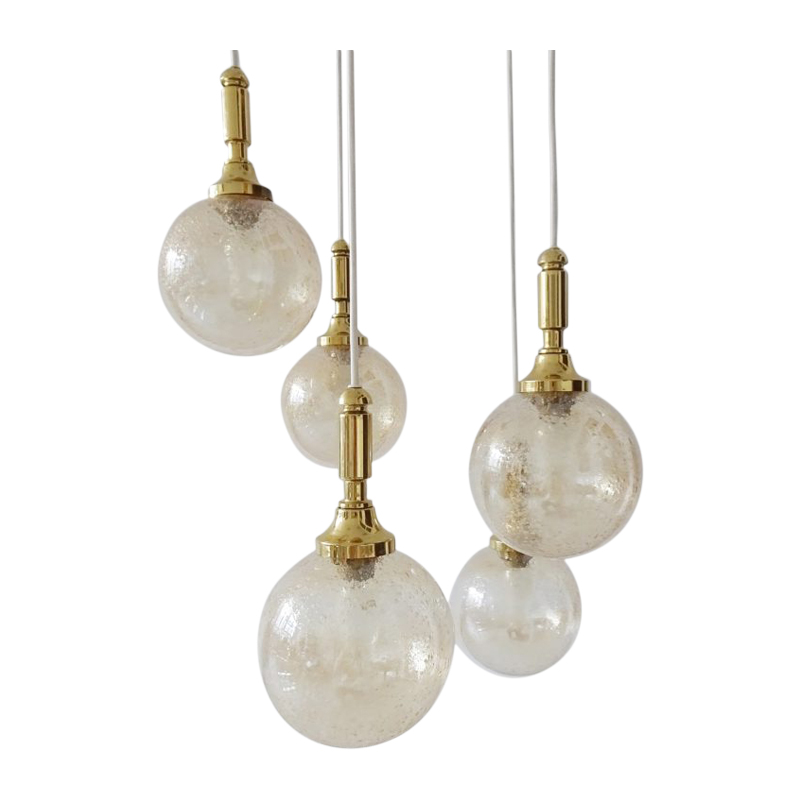The image features five ornate hanging light fixtures, each designed with a frosted, imperfect glass bulb that appears handcrafted or glass-blown. These bulbs are mounted on a golden metal base and are suspended at various heights from thick white cords attached to the ceiling. The light fixtures' arrangement at different levels adds an intentional aesthetic touch, while the backdrop is a plain, empty white, emphasizing the elegant simplicity and decorative nature of the lights.